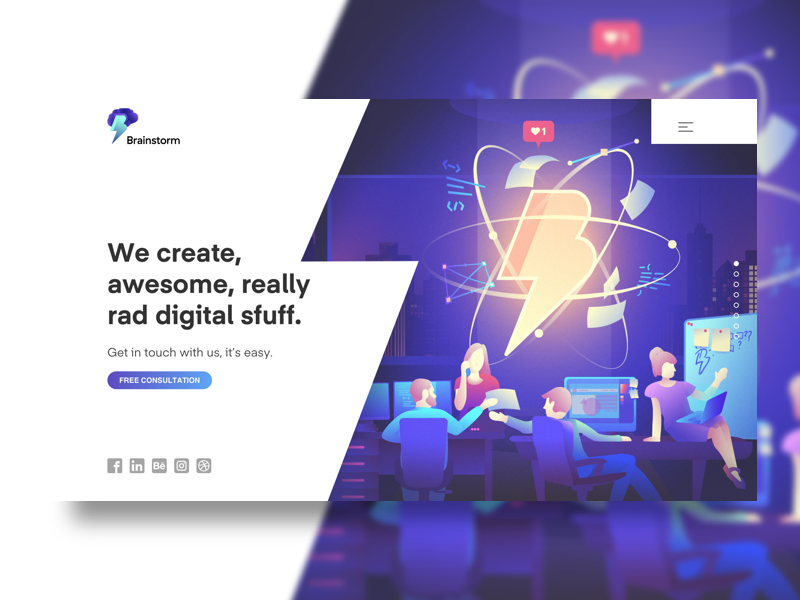In this image, we're presented with a vibrant, cartoon-style depiction of an office setting, exuding a relaxed and casual atmosphere. Dominating the right-hand side of the frame, there is a purplish background that covers approximately three-quarters of the image. Layered into this purplish hue is a blurred version of the same scene, creating an almost seamless overlay effect.

In the foreground, four cartoon-style characters are depicted, suggesting an environment teeming with creativity and collaboration. Prominently featured is a symbol reminiscent of an atom, akin to illustrations found in science magazines. This atom-like symbol contains a central letter "B" followed by a squiggly line resembling the letters "BS."

On the left-hand side, near the same atom symbol, the word "brainstorm" is prominently displayed. Accompanying text reads, "We create awesome, really rad digital stuff. Get in touch with us," portraying a vibrant invitation to engage with the creative team. Overall, the image conveys a dynamic, playful, and approachable atmosphere, typical of a modern digital workspace.